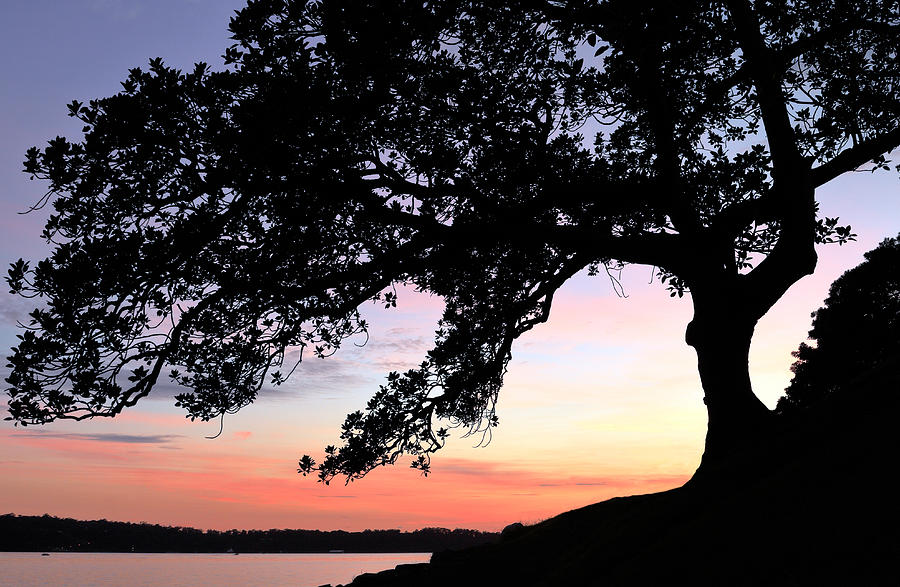The photograph captures a stunning natural scenery at sunset, presenting a vibrant sky transitioning through a spectrum of colors—deep blue at the top, fading into pinks, oranges, and finally yellows near the horizon. The foreground features a large tree in full silhouette, positioned in the bottom right corner. The tree’s extensive branches and leaves stretch across the image, creating intricate patterns against the multi-colored sunset sky. Below the silhouette of the tree, the image depicts a body of water on the lower left side, reflecting some of the sky's hues. Beyond this, more vegetation forms a darkened, silhouetted line. A few dark gray-purple clouds streak across the sky, adding depth to the serene, picturesque landscape. The overall composition emphasizes the striking contrast between the silhouetted natural elements and the vividly colored sunset.